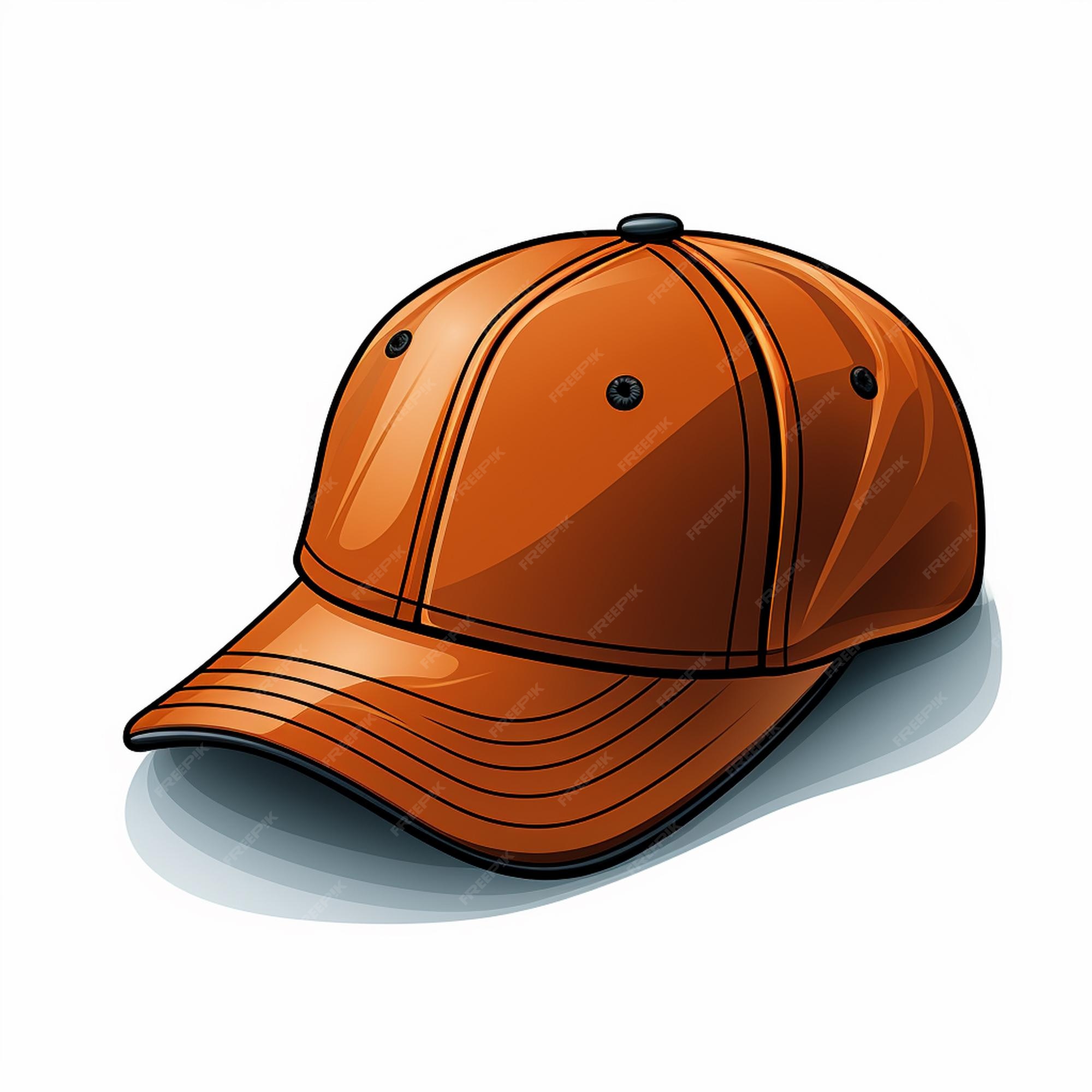This digital graphic depicts an orange ball cap, which appears to be floating against a stark white backdrop. The rendering of the hat showcases various shades of reds and oranges, simulating lighting effects that create a sense of depth and realism. The cap is oriented in a slightly overhead, head-on perspective, allowing a clear view of the entire brim, which is bordered in black with four black lines accentuating its structure. The top of the hat features black air holes within the visible segments and a central black button. Below, the shadow of the hat shows layers of grays and dark shades, reinforcing the lighting from above. The image includes a subtle, repetitive "Free Pick" watermark that runs diagonally across the hat, lending a textured appearance.